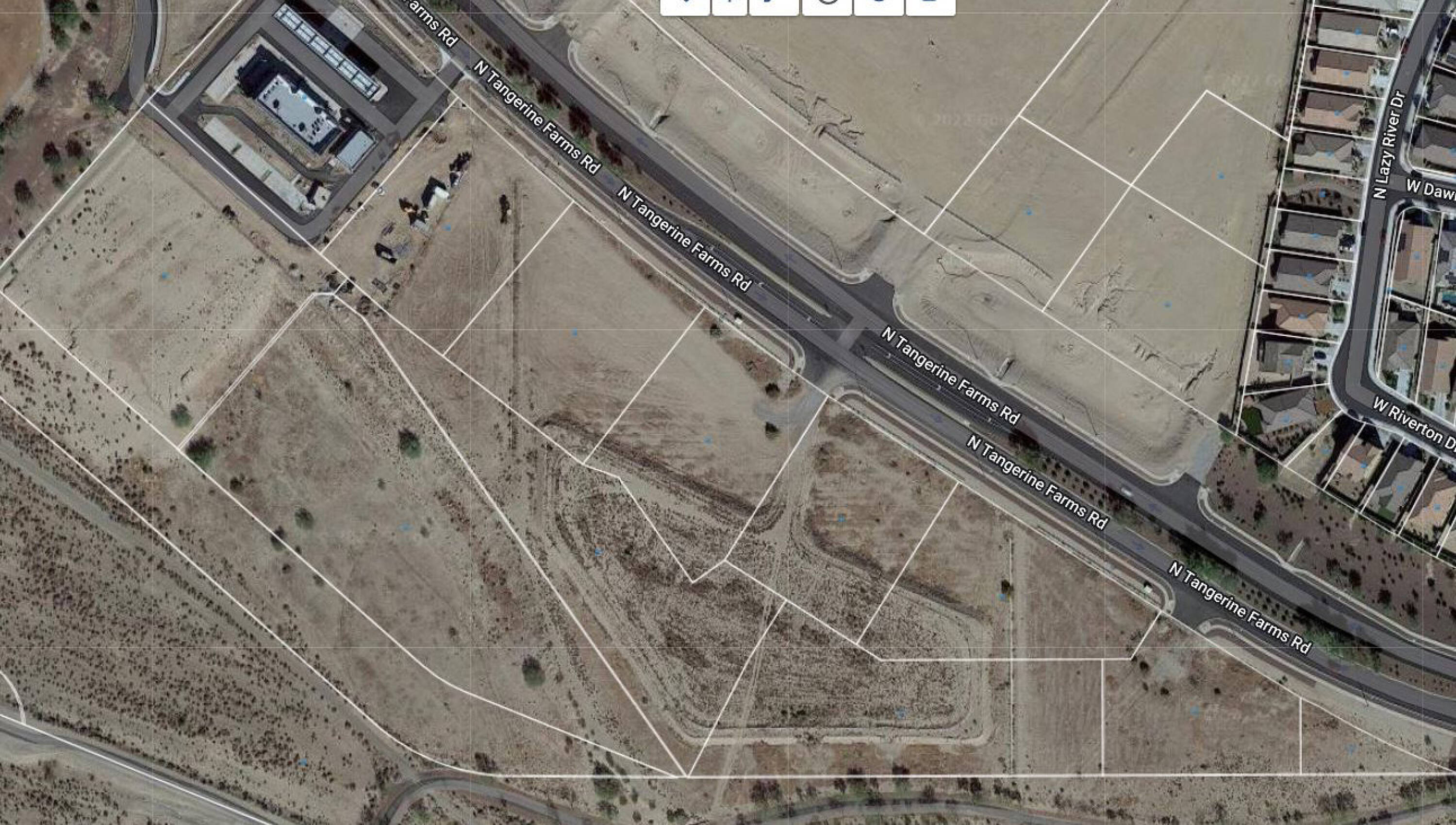This is a detailed aerial, bird's eye view photograph of a suburban intersection in a deserty area. The image prominently displays North Tangerine Farms Road, labeled in white text superimposed directly on the road, stretching diagonally from the lower right to near the upper left corner of the photograph. Another road in the upper right portion of the photo is identified as West Riverfront Drive, with additional roads such as North Lazy River Drive and West Dawn also visible. The upper portion of the image highlights a densely packed subdivision with suburban houses, whereas the majority of the scene features barren, vacant land with minimal vegetation. Near the upper left corner of the photograph, there is a building with people emerging from cars, despite the high elevation of the shot.